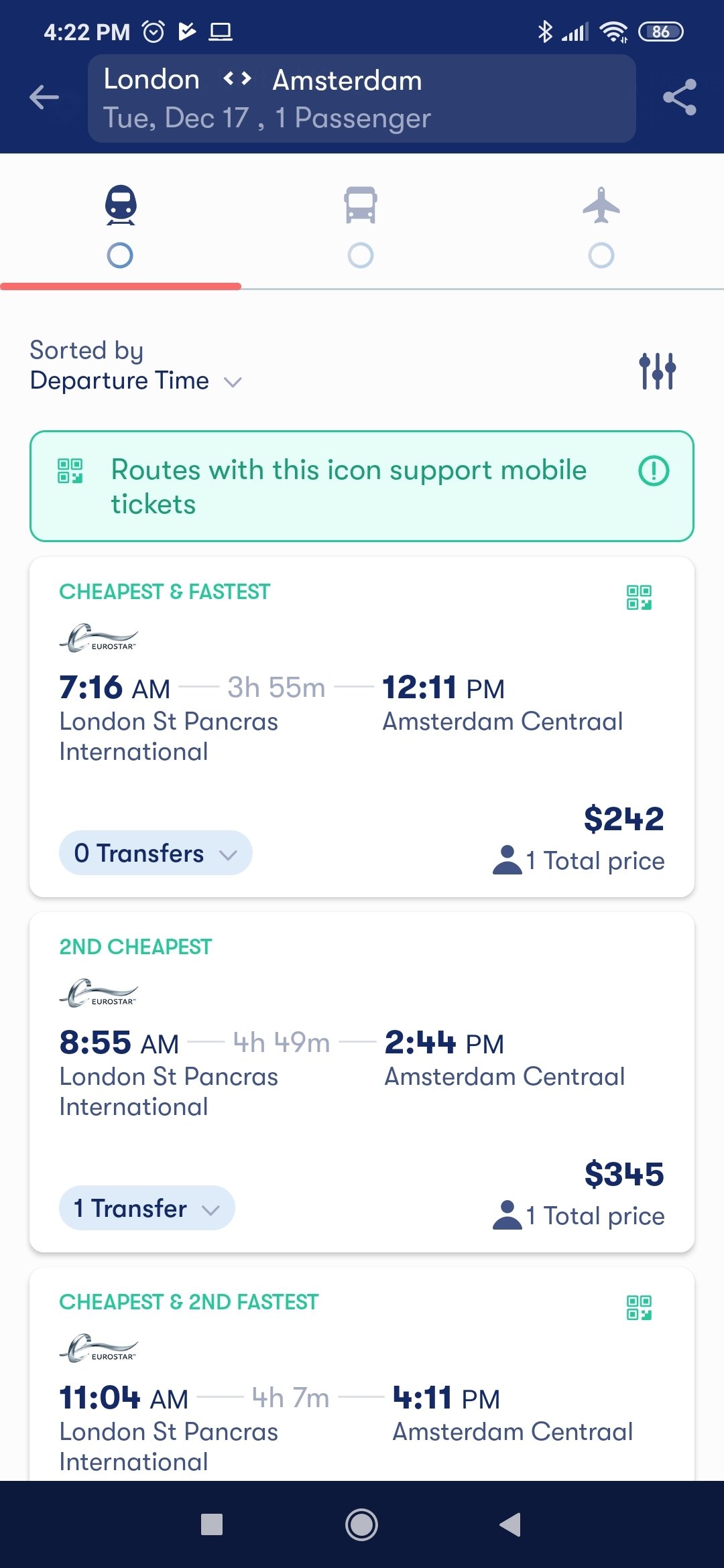This image, captured on an iPhone screen, presents travel information for a route between London and Amsterdam. The screenshot features a sophisticated interface with a dark blue header displaying the cities 'London' and 'Amsterdam,' along with the current time, which is 4:22, and a battery life indicator showing 86%. Below, it mentions the date 'Tuesday, December 17th' and specifies 'One passenger' with a left-pointing arrow. Icons suggest options for travel by car, bus, or plane, with 'car' underlined in orange. 

The interface allows sorting by departure time and highlights important travel information. A green box notes that routes with the specified icon support mobile tickets, accompanied by green lettering designating 'cheapest' and 'fastest' options. 

There's a list of routes from 'London Street, Pancos International' to 'Amsterdam Central.' The first option is stated as having no transfers, emphasizing convenience with a highlighted departure time. The second option from the same departure to destination points involves one transfer, marked in a blue circular box. Despite being the second cheapest, it offers a later departure. 

Another option is noted as the 'cheapest and second fastest,' though the extended travel time is significantly longer and part of the text is cut off, leaving the number of transfers unclear. This detailed interface offers a comprehensive comparison for travelers choosing the best route between London and Amsterdam.